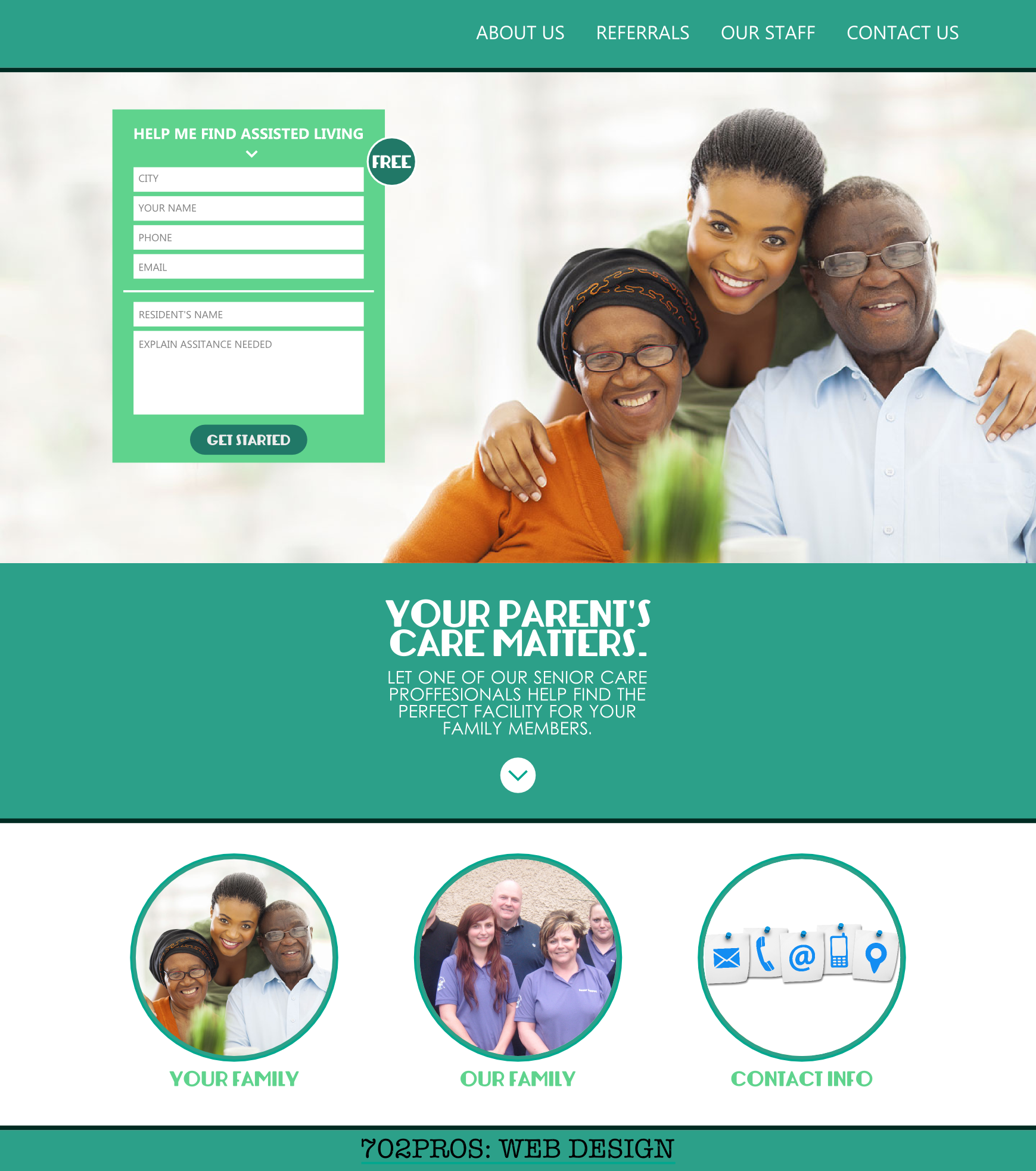This screenshot captures a webpage dedicated to senior care services. At the top of the page, a Kelly green banner with white text displays navigation options: "About Us," "Referrals," "Our Staff," and "Contact Us." 

Below the banner, a heartwarming photo features three African American individuals. Sitting on the left is an elderly woman, likely in her 70s, wearing a black turban, orange shirt, and glasses. Beside her, an elderly man, also appearing to be in his 70s, is dressed in a light blue button-down collared shirt. Between them, a young woman stands smiling, her head positioned lovingly between the older couple.

To the left of the photo, there is a form titled "Help Me Find Assisted Living," which includes dropdown menus and fields for "City," "Your Name," "Phone," "Email," "Residence Name," and "Explain Assistance Needed." At the bottom of the form, a prominent "Get Started" button invites users to take the next step.

Beneath the image of the three family members, against a green background, there's a message in white text that reads: "Your Parents' Care Matters. Let one of our senior care professionals help find the perfect facility for your family members."